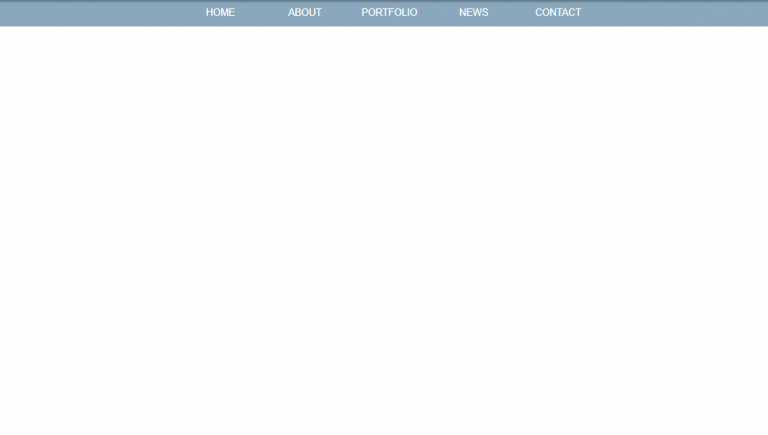The image showcases a blank webpage with a pure white background. The only content present is a horizontally-arranged menu bar across the top of the page. This menu bar features a gradient of light blue transitioning to a darker blue at the top edge. The menu items "Home," "About," "Portfolio," "News," and "Contact" are displayed in evenly spaced white text. The rest of the webpage is completely empty, suggesting it is either not working or has not loaded properly. There is no additional content or visual elements beyond the menu bar.